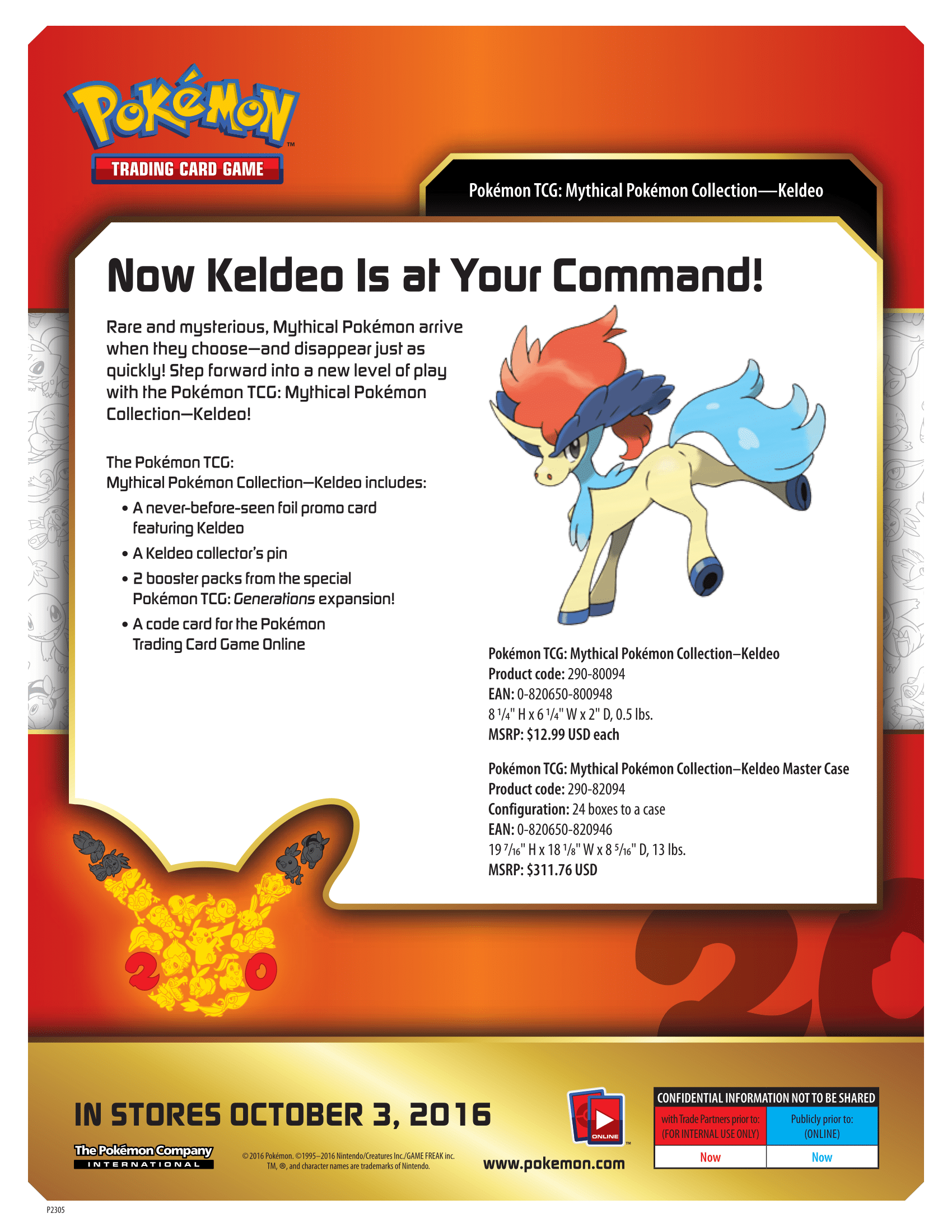The poster for the Pokémon Trading Card Game (TCG) features a striking design centered around the Mythical Pokémon Collection with a focus on Keldeo. At the top, bold text introduces Keldeo, a specific Pokémon, heralding its arrival with the phrase, "Keldeo is at your command." The illustration depicts Keldeo, which resembles a small pony with a blue, poofy tail and a distinctive blue and red mane. The Pokémon exudes a youthful, lean, and spirited demeanor, captured mid-action as it bucks its back legs.

Below this vibrant representation, the poster provides details about Keldeo. It describes the arrival of rare and mysterious mythical Pokémon, emphasizing their unique appearance and transient nature: "Rare and mysterious mythical Pokémon arrive when they choose, then disappear just as quickly. Step forward to a new level of play with the Pokémon TCG." 

Further down, the poster highlights the exclusive inclusions of this collection, stating, "Keldeo includes a never-before-seen foil promo card featuring Keldeo." This promise of unique content adds an element of exclusivity and excitement for collectors and players alike.

The bottom section of the poster features an artful image of Pikachu, designed in a creative mosaic style. This artsy Pikachu is composed of numerous smaller Pikachu figures, creatively arranged to form a larger Pikachu face, adding a unique artistic touch to the overall design of the poster.